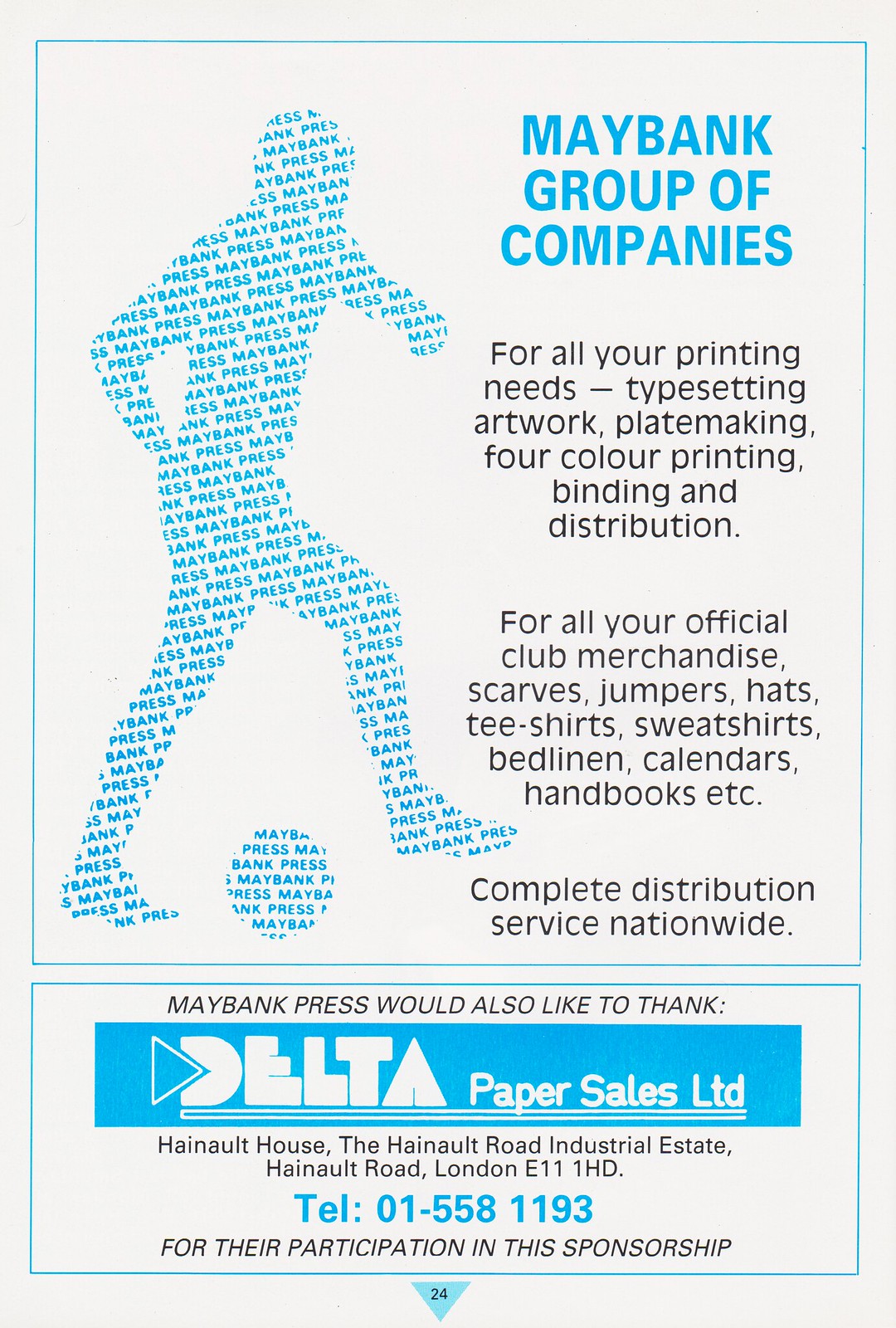This portrait-oriented flyer, potentially a magazine page, features a light gray background with a detailed promotional design. Dominating the top section is a tall rectangle outlined in light blue, containing an eye-catching graphic of a person kicking a soccer ball. This illustration is uniquely composed of bright blue, all-capital letters that repeatedly spell out "Maybank Press," arranged diagonally.

To the upper right of this graphic, in all-capital blue letters, it reads "MAYBANK GROUP OF COMPANIES." Below this header, the text details the services offered, including "for all your printing needs, typesetting, artwork, plate making, four-color printing, binding, and distribution." It also advertises merchandise solutions for clubs, listing various items like scarves, jumpers, hats, t-shirts, sweatshirts, bed linen, calendars, and handbooks, along with a complete nationwide distribution service.

Beneath this, there is a wide rectangle also outlined in light blue, where "Maybank Press" extends its gratitude to Delta Paper Sales Limited for their sponsorship. The address and a phone number for Delta Paper Sales Limited are provided, located at Hainaut House, the Hainaut Road Industrial Estate, Hainaut Road, London E11, 1HD. This well-organized poster, marked by its strategic layout and professional color scheme of gray, blue, black, and white, exudes the polished essence of a magazine advertisement.